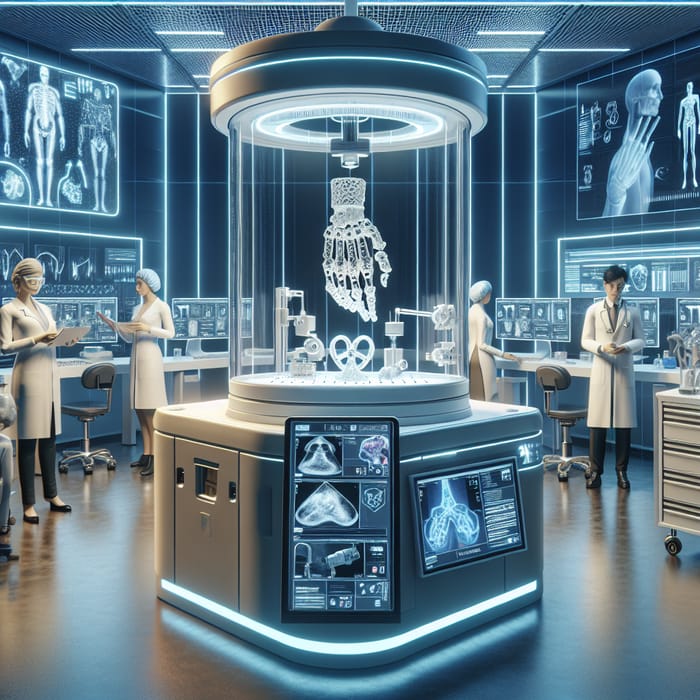The image depicts a high-tech, computer-generated indoor scene set in a robotics laboratory. The environment is illuminated by bright ceiling lights and is dominated by a bluish hue, adding to its futuristic ambiance. Central to the image is a sophisticated machine that resembles a tank, housing what appears to be a skeletal hand, possibly robotic in nature. Surrounding this primary apparatus, several digital screens are visible, positioned on the top right and top left, and there are additional computer monitors near white desks on both sides. Black chairs complement the workspace setup, while scientists, including a man with black hair, stand on either side, contributing to the meticulous and organized atmosphere. The detailed background is filled with advanced equipment, suggesting an environment ripe with innovation and cutting-edge technology, akin to a scene from a highly detailed video game or digital artwork.